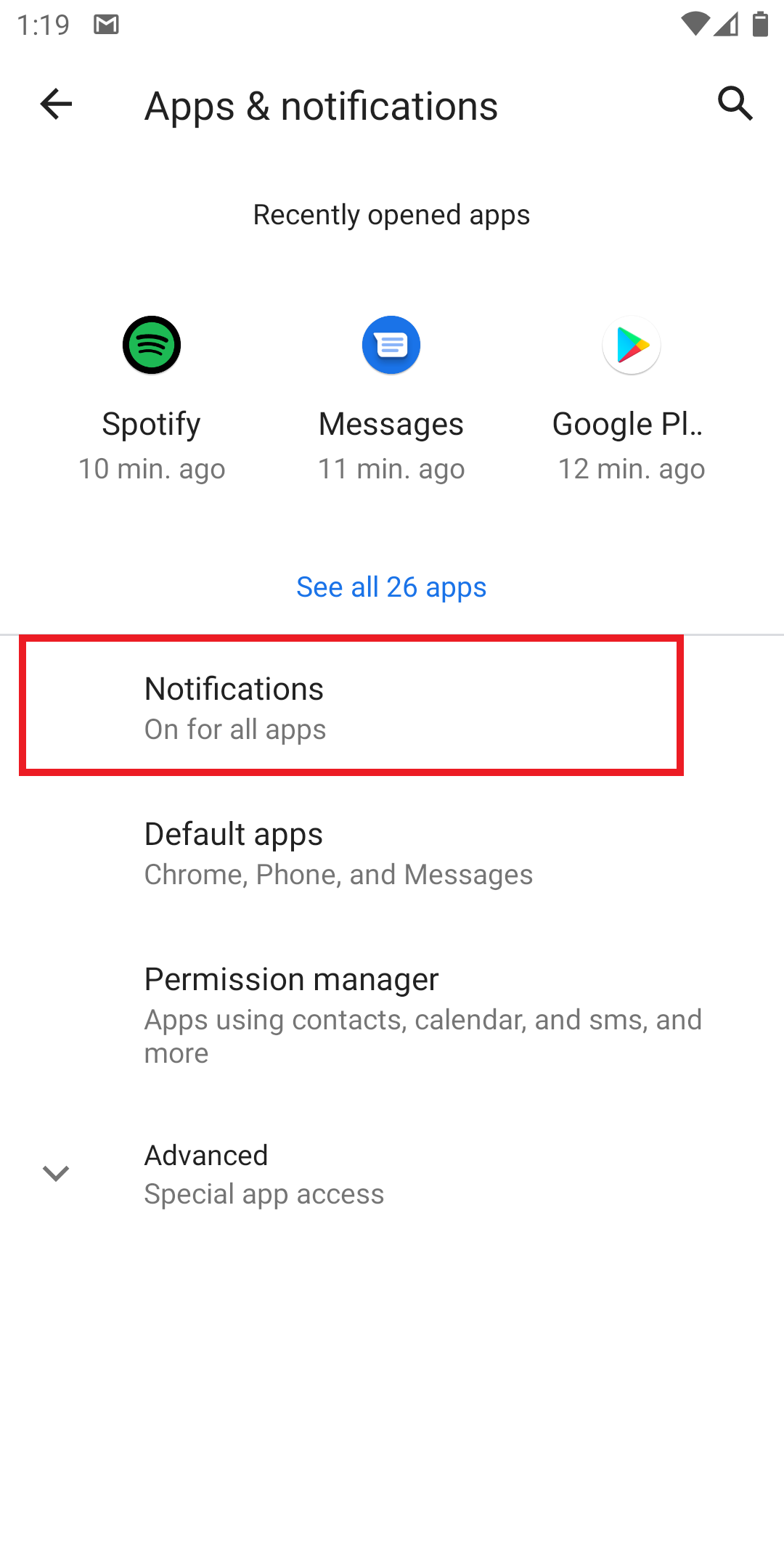The upper portion of the screen displays a clean, white background with the time indicated in grey as "1:119". Positioned next to this is a grey square with a white "M", suggesting the Gmail app. The Wi-Fi icon appears grey, indicating a strong connection, and the reception bars are mostly grey with a hint of white, denoting decent phone service. The battery icon is predominantly grey, signifying a nearly full charge.

Below this section, on the left side, there's a black arrow pointing right, accompanied by the text "Apps & notifications". Next to it, there's a black magnifying glass icon. Directly below, centrally placed, is a header titled "Recently opened apps". This section features three circular icons: 
1. The first icon is green and black, representing Spotify, which was opened 10 minutes ago.
2. The second icon is blue and white, representing Messages, opened 11 minutes ago.
3. The third icon is white with a colorful triangle made up of red, yellow, green, and blue elements, representing Google PL, opened 12 minutes ago.

Following these icons, in blue text, there's an option to "See all 26 apps". A thin grey line runs horizontally across the screen, separating the sections.

Next, in black text, the section titled "Notifications" appears, followed by the subheader "All on for 4 apps" encased in a red box, suggesting it might be selected or highlighted.

Further down, there is a white space followed by a list detailing the 4 apps, which includes "Chrome", "Phone", and "Messages". Another stretch of white space is seen next.

Finally, in black text, a section titled "Permission Manager" outlines "Apps using contacts, calendar, SMS, and more", with a subsequent section marked "Advanced Special app access".